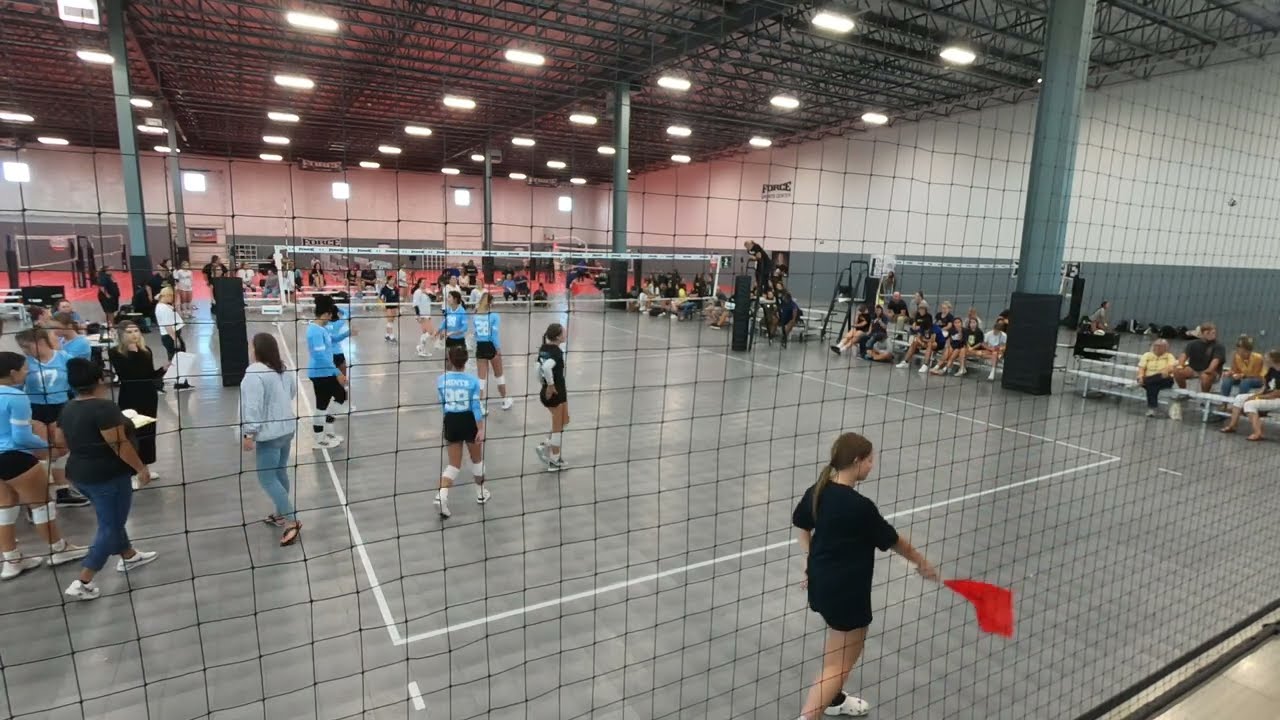The image is a detailed photograph taken inside a large gymnasium during a volleyball tournament. It features a volleyball court prominently on the right-hand side of the building, with an open area on the left suggesting there may be another court not fully visible. The gym has white walls with a gray lower section, and the ceiling is equipped with bright overhead lights supported by steel grates and beams—three on the right and two on the left.

The court is surrounded by netting, presumably to contain the volleyball. On the right side, there are small, removable white bleachers with spectators. There are more people positioned on the left and in the background, though their activities are unclear from the image. 

The players on one side are mainly wearing light blue or black and white long-sleeve shirts paired with black shorts, indicating the team colors. A referee, distinguished by a black outfit and holding a red flag, is positioned closest to the viewers. Additionally, several coaches and possibly some parents are seen interacting with the players, suggesting a timeout situation. Far in the distance, a red track is visible at the top end of the building, adding depth to the sports complex environment.